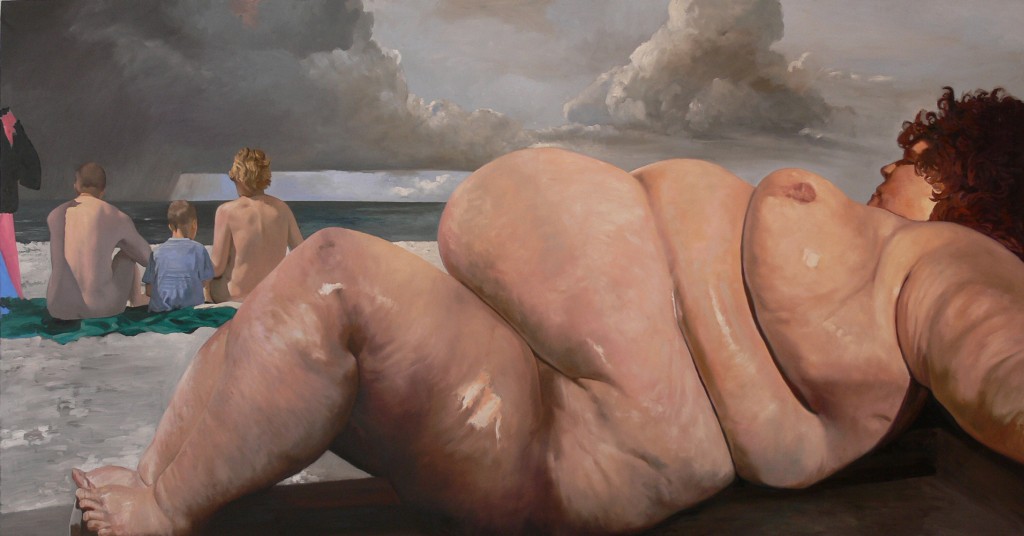The painting depicts an extremely obese, nude woman with long, dark curly hair, lying on her back on the beach with her knees bent and her arms spread out beside her. She has a shiny, almost unrealistic skin tone, and her head is turned slightly to her right as she looks towards a group of people on her left. These people are sitting on a green picnic blanket and seem to be looking out towards the ocean. Among them, there is a man, a woman, and a child wearing a blue shirt, potentially indicating a family unit. Additionally, two of the adults appear to be nude. In the background, the horizon shows a dark, moody sea, while the sky above is filled with dark grey clouds on the top left and smaller, lighter grey clouds on the top right. The beach sand on the left side of the painting is a light grey-brownish color, adding to the overall somber and tranquil atmosphere of the scene.